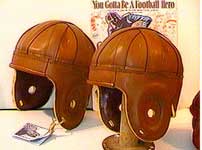The image depicts two vintage brown leather football helmets with a mix of dark and light brown tones, resting on a white table. Both helmets are old-fashioned, devoid of modern face guards, and equipped with ear flaps. The helmet on the right is propped up on a wooden pole, while the one on the left leans against something in the background. A notable feature is a cartoonish illustration of a football player on top of the right helmet, accompanying text that reads, "You gotta be a football hero." Additionally, there is a small note connected to the right flap of the left helmet, though the image on it is unclear. The overall scene is animated and somewhat cartoon-like. The background is predominantly white, except for this vintage advertisement.